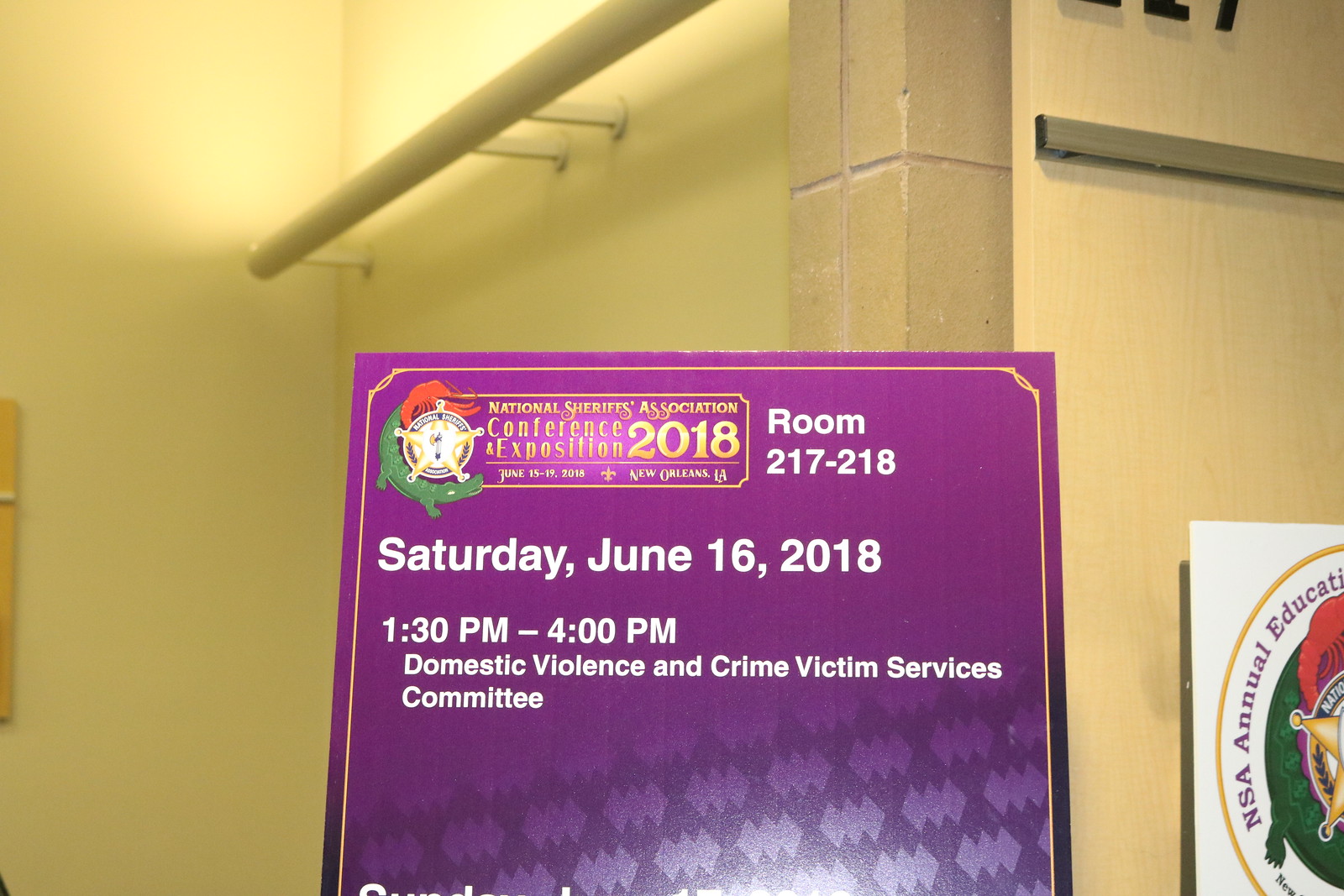The image is a color photograph taken in landscape orientation inside a conference hall with beige and wooden walls. The main subject is a vertical, purple information banner prominently displayed in the center, though partially cut off at the bottom. This banner features a darker purple section at the bottom adorned with a repeating pattern of three interconnected diamonds. Across the top, white lettering reads details of an event: "Saturday, June 16, 2018, 1:30 to 4 p.m. Domestic Violence and Crime Victim Services Committee.” In the top left corner, a gold-bordered logo reads, "National Sheriffs Association Conference and Exposition 2018, New Orleans, Louisiana," with additional text indicating "Room 217 to 218." The sheriff's badge logo, featuring green and red accents, is also visible beside this text. To the right of the main banner is another partially cut-off poster, similarly themed, that also displays a Sheriff's Association logo. The setting includes racks, shelves, and black lighting, suggesting an interior conference environment.